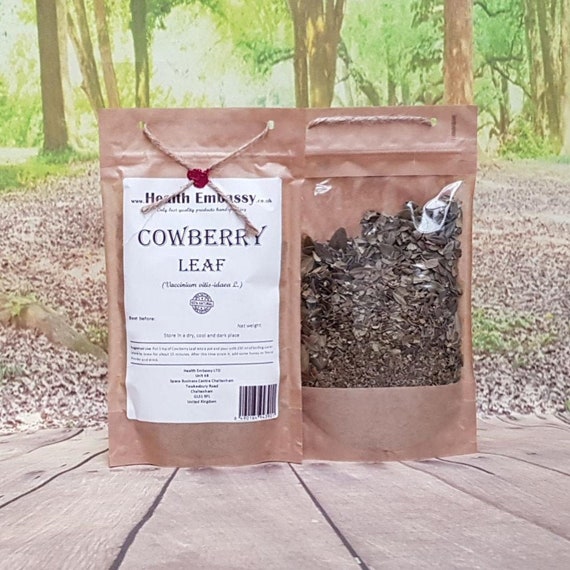The image depicts a serene, sunlit forest scene with a backdrop of bright green leaves and brown tree trunks occupying the top third of the picture. The middle section features a brown ground scattered with pebbles and patches of greenery. The bottom third shows a wooden decked area, where two brown packages labeled "Cowberry Leaf" from the brand "Health Embassy" are prominently displayed. The package on the left shows the front, featuring detailed labeling, including a prominent "Cowberry Leaf" text and additional instructions and descriptions. The package on the right reveals the back, showcasing a transparent window through which the contents—black and gray seeds—are visible. A barcode can also be seen on the back package. This juxtaposition of natural elements and product packaging evokes a sense of organic authenticity and wellness.